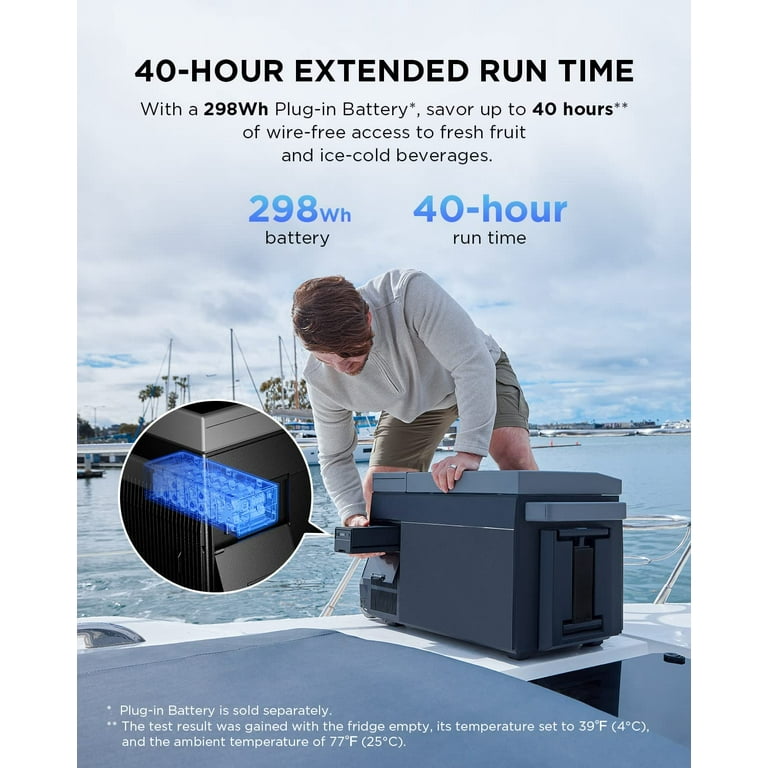The rectangular image, approximately six inches high and four to five inches wide, showcases a detailed advertisement for a portable refrigerator set on a sailboat. The background features a light gray cloudy sky with hints of blue, and below that is a harbor with blue water and some sailboats. In the foreground, a Caucasian man is bent over a black and gray portable refrigerator, reaching out with his right hand to pull out a blue ice tray from the appliance. This close-up action is emphasized with an insert highlighting the ice tray. 

Bold black text at the top center of the image reads, "40-hour extended run time with a 298 WH plug-in battery." Further down in blue and black text, it states, "298 WH battery" and "40-hour run time," along with the phrase, "Save up to 40 hours of wire-free access to fresh fruit and ice-cold beverages." An asterisk at the bottom notes that the plug-in battery is sold separately, while another asterisk specifies that this test result was achieved with the fridge empty, set to 39 degrees Fahrenheit (4 degrees Celsius), and an ambient temperature of 77 degrees Fahrenheit (25 degrees Celsius). 

The scene is designed to showcase the utility and convenience of the portable refrigerator in boating conditions, emphasizing its extended battery life and ability to keep contents cold.